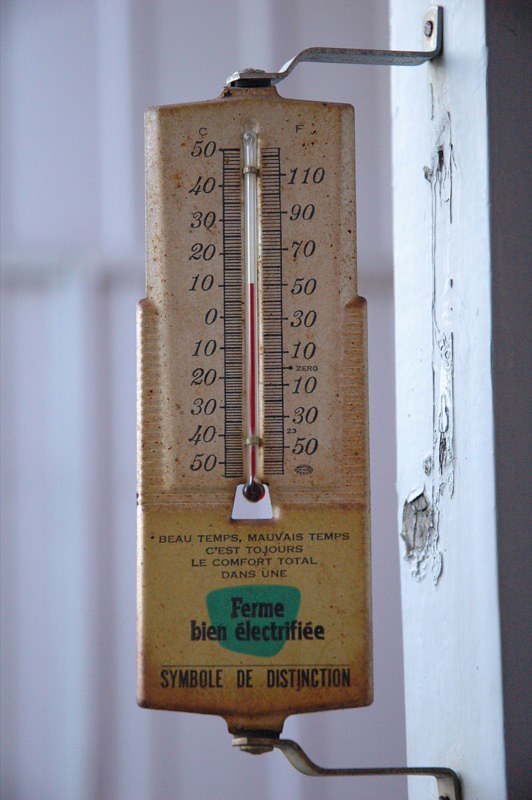A close-up photograph of an old and dirty thermostat, displaying a temperature of 10°C (50°F). The device appears worn out, with visible dirt and grime on its surface, highlighting its age and frequent use. The image captures the intricate details of the thermometer's dial and markings, emphasizing its vintage and utilitarian appearance.